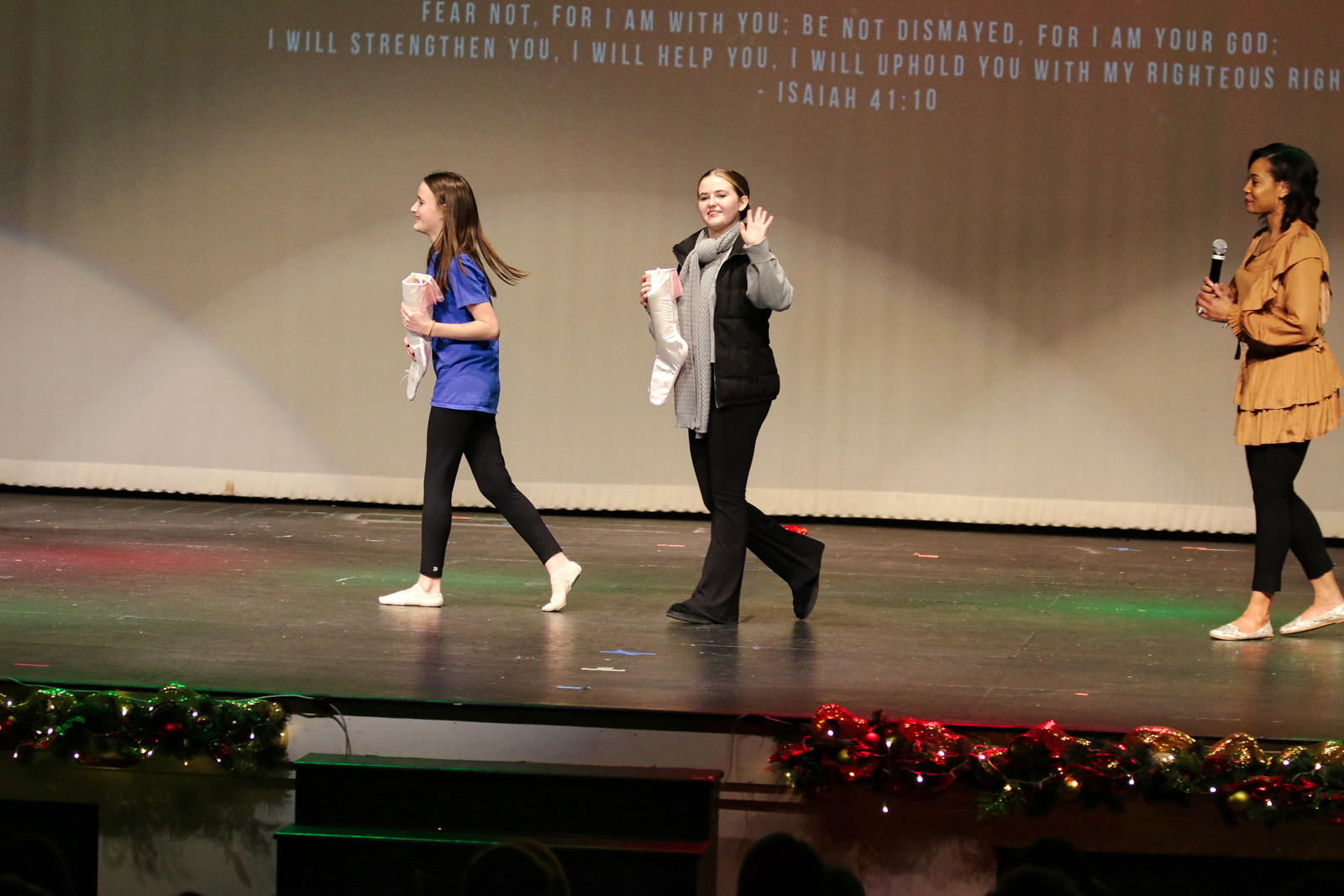The photograph, approximately six inches wide by four inches tall, depicts a stage setting likely from a 2024 Christmas pageant. Three females are featured, two of whom appear to be teenagers. They are walking across the stage from right to left. The foreground figure, a Caucasian girl with long brown hair, is dressed in a short-sleeved blue shirt, black pants, and white shoes. She carries a pale-colored stuffed animal. Behind her, another Caucasian girl with sandy blonde hair pulled back in a bun wears a black puffer vest, black pants, a gray long-sleeve shirt, and a gray scarf, carrying a white stuffed animal while smiling and waving at the audience. Further back, a woman of African descent with tan skin and black hair holds a microphone in both hands. She wears a mustard-yellow ruffled tunic, black leggings, and white shoes. 

The background reveals a light-colored curtain or screen onto which a Bible verse from Isaiah 41:10 is projected in white text: "Fear not, for I am with you; be not dismayed, for I am your God. I will strengthen you, I will help you, I will uphold you with my righteous right." Three overlapping spotlights create arcs of red, green, and blue across the horizontal plane. The stage itself features colorful splotches, possibly from painted designs or additional lighting effects, and is adorned with Christmas decorations. On the right side are red poinsettias, and on the left are conifer branches with gold, red, and blue Christmas ornaments. The stage ends with steps leading downwards, black and green in color, with a white backdrop.